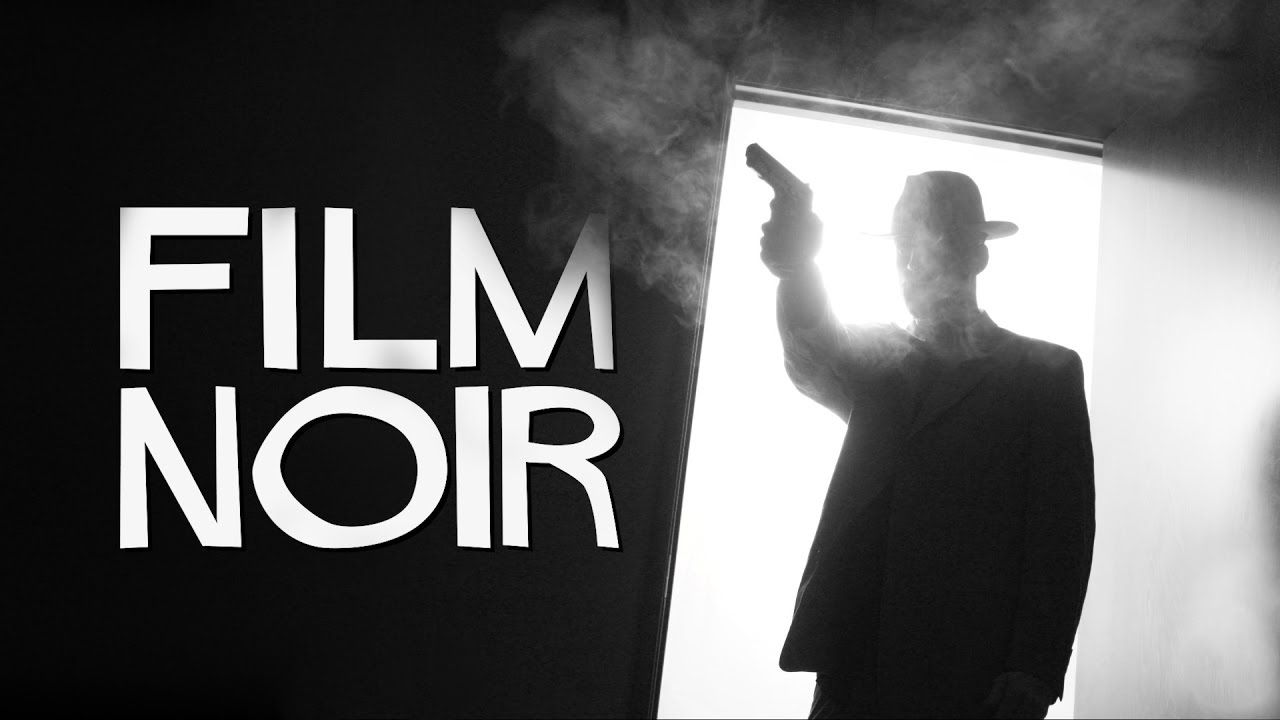The horizontally aligned rectangular black and white photo features a stark contrast between darkness and light. The left side of the image is completely black, with large, bold, all-caps white letters centered vertically, reading "FILM NOIR." Adjacent to this text, on the right side of the image, an open doorway emits a bright, almost blinding light that envelops the scene in a smoky haze. 

In front of this illuminated doorway stands the silhouette of a man facing us. His features are obscured by the interplay of light and smoke, but he is discernible by his wide-brimmed fedora and dark attire, which includes a black suit or jacket and dark pants. The man's right arm is extended forward, towards the upper left side of the image, holding a black handgun. The smoke, presumably from a recent gunshot, swirls around him, adding to the mysterious ambiance. The stark white of the light and smoke provide a dramatic backdrop against his dark silhouette, enhancing the film noir aesthetic of the scene.